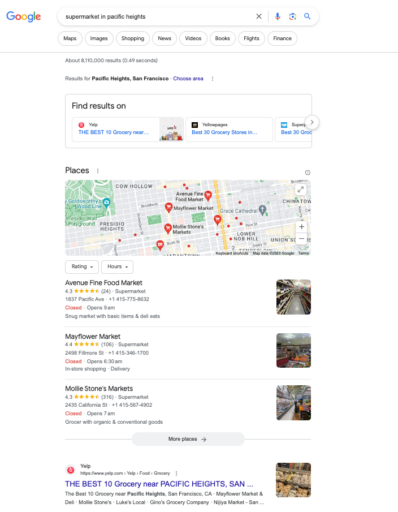The image is a blurry screenshot of a mobile-oriented search results page on Google. At the top center, there is a prominent Google search bar featuring the Google logo on the left. On the right side of the search bar, there are three icons: a microphone, a colored circle, and a magnifying glass. Just below the search bar are bubble-style headings labeled Maps, Images, Shopping, News, Videos, Books, Flights, and Finance.

Beneath these headings, the results section begins with a white text box indicating where to find relevant information. The section titled "Places" follows, showcasing a street map with red markers indicating various locations. Some of the identifiable areas on the map include Mayflower Market and Lowe's Knob Hill.

Below the map, there are three market advertisements displayed in a horizontal strip against a white background, each accompanied by an image of the respective market on the right-hand side. These markets are Avenue Fine Food Market, Mayflower Market, and Mobile Stones Market. Under this strip, a gray button is available, inviting users to click and discover more places.

Further down, there is a listing from Yelp titled "The Best Ten Grocery Stores near Pacific Heights Sand," featuring a photograph of a market on the right-hand side with descriptive black text beneath it. This text is clickable, leading to the Yelp page for more detailed information.